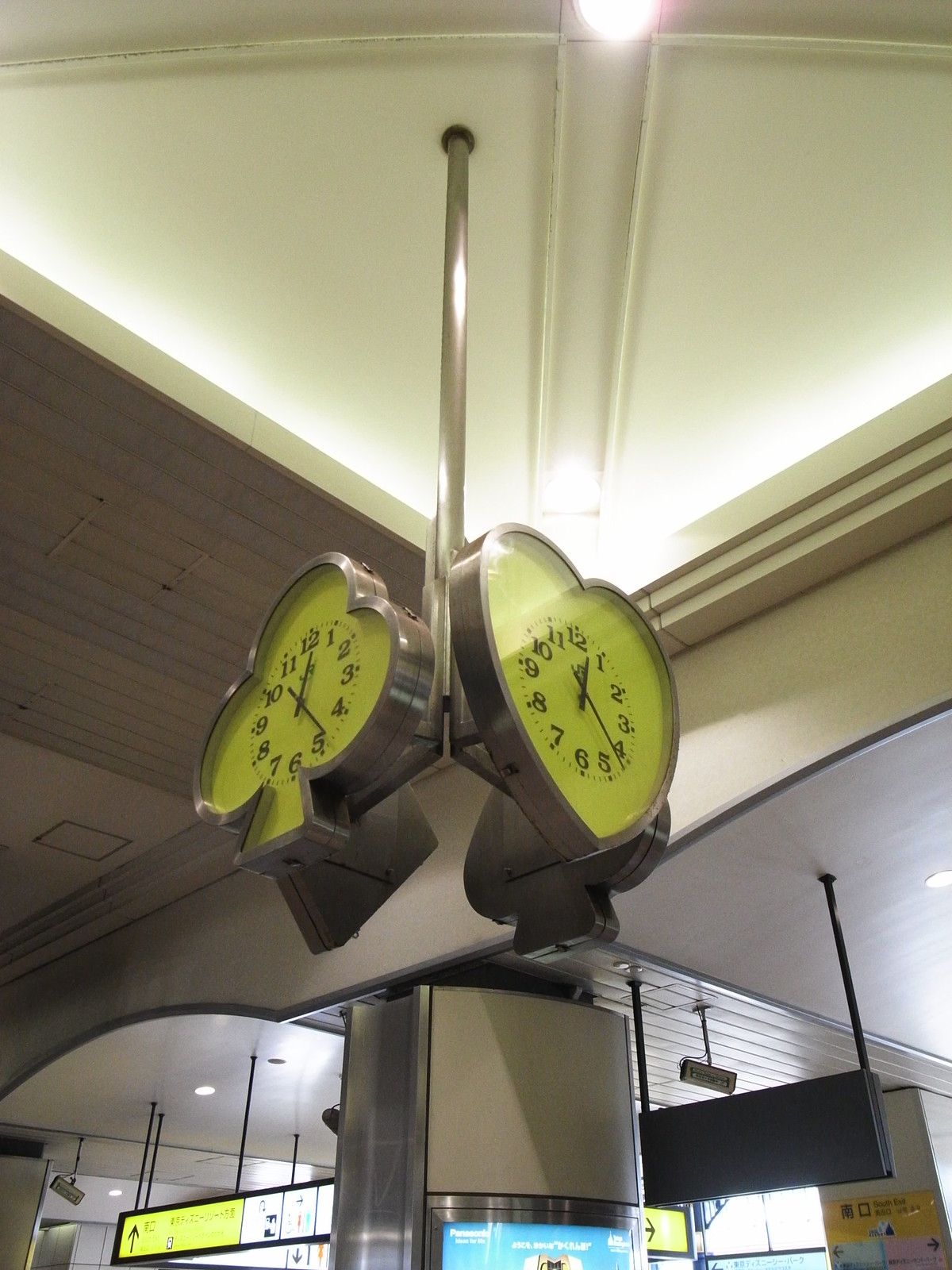This photograph captures a unique installation of four clocks, each inspired by the suits of playing cards, hanging from the ceiling. Each clock features a metallic outer layer with a vibrant yellow face. The clocks, facing different directions, depict the four card suits: a club facing the bottom left, a heart facing the bottom right, a spade facing the upper right, and a diamond facing the upper left. The background suggests that this installation is located in a transit hub, potentially a train station or an airport, as indicated by the visible signage. Notably, all four clocks display the same time, adding a cohesive and whimsical touch to this creative display.